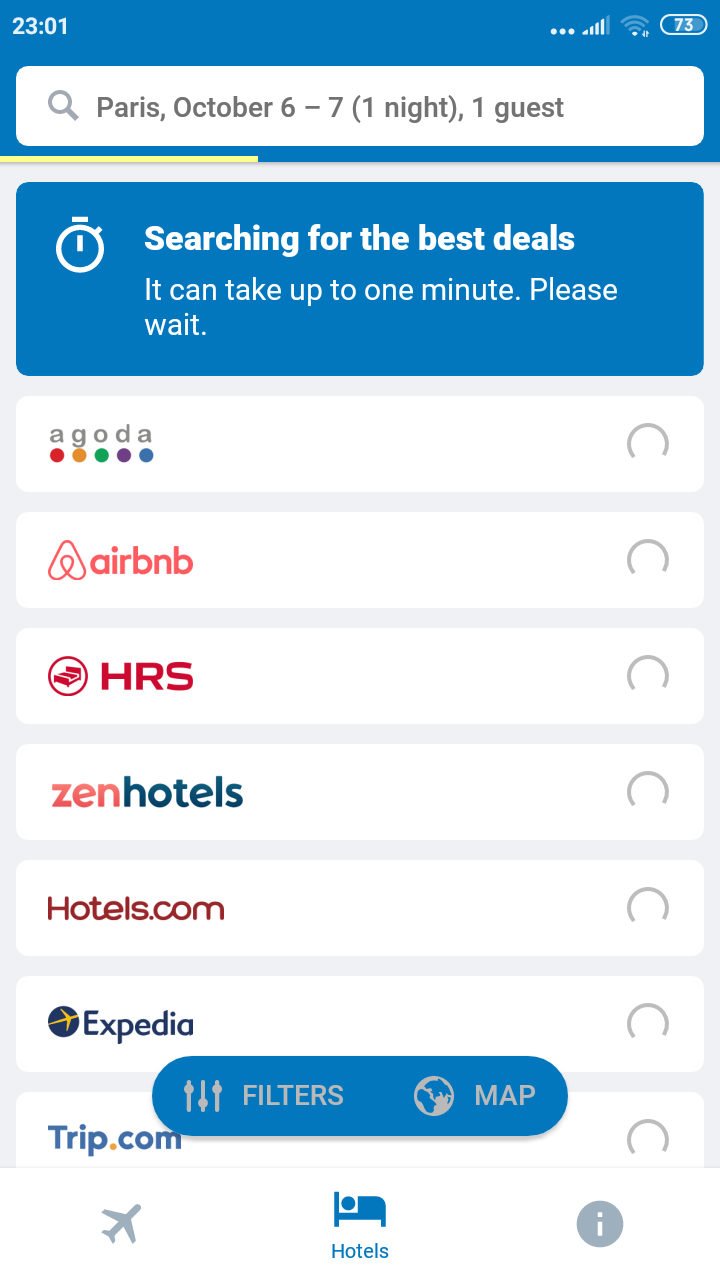The image depicts a mobile app interface related to travel accommodation booking. In the upper left corner, set against a blue border, the time is displayed as "23:01" in white font. On the upper right, there are indicators for data connection, Wi-Fi, and a battery icon within a white oval showing the number "73". Beneath these indicators, a white search bar displays the input "Paris, October 6-7, one night, one guest."

Further down, a blue text box occupies a central area with the message "Searching for best deals. It can take up to one minute, please wait" accompanied by a small stopwatch icon on the left. Below this, several categories are listed including Agoda, Airbnb, HRS, Zen Hotels, Hotels.com, Expedia, and Trip.com.

A blue pop-up labeled "Filters" is next to another option "Map" in gray. At the bottom, there are icons for an airplane, a hotel, and an information "i" symbol. The hotel icon, which resembles a bed with a person sleeping in it, is highlighted in blue, indicating that the current page is related to hotel bookings.